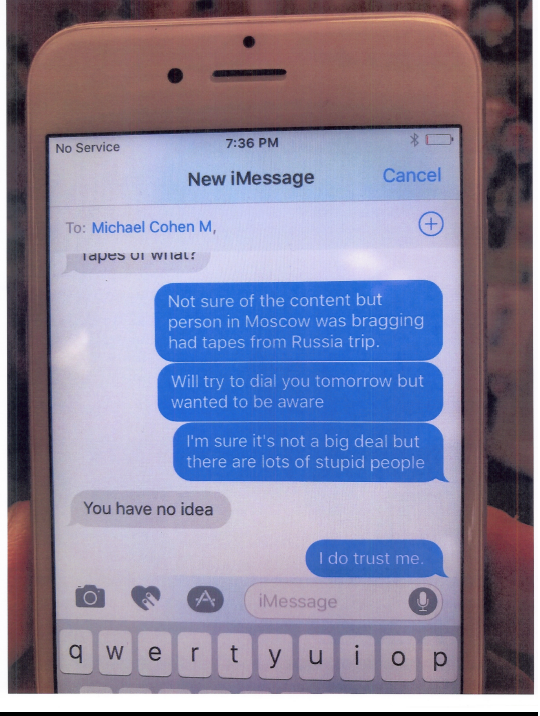This is a detailed color photograph of an iPhone screen displaying an iMessage conversation. The iPhone has a white frame, and at the top of the screen, it shows "No Service" and a time of 7:36 p.m. The battery icon is displayed in white and red, indicating it is low. Below this status bar, the screen indicates a new iMessage to "Michael Cohen M" with a blue 'Cancel' option adjacent to it.

The text message conversation features prominently in the image. The top message, in a blue bubble with white text, reads: "Not sure of the content that person in Moscow was bragging. Had tapes from Russia trip. Will try to dial you tomorrow but wanted to be aware. I'm sure it's not a big deal but there are lots of stupid people." This message is stacked in a series of rectangular blue bubbles with rounded edges. 

Following this, there is a gray bubble on the left with black text that says, "You have no idea." In response, a smaller blue bubble on the right with white text states, "I do trust me."

At the very bottom of the screen, the iPhone's standard navigation bar is visible, showing icons for the camera, heart, and message input area where it says "iMessage," along with the top portion of the keyboard.